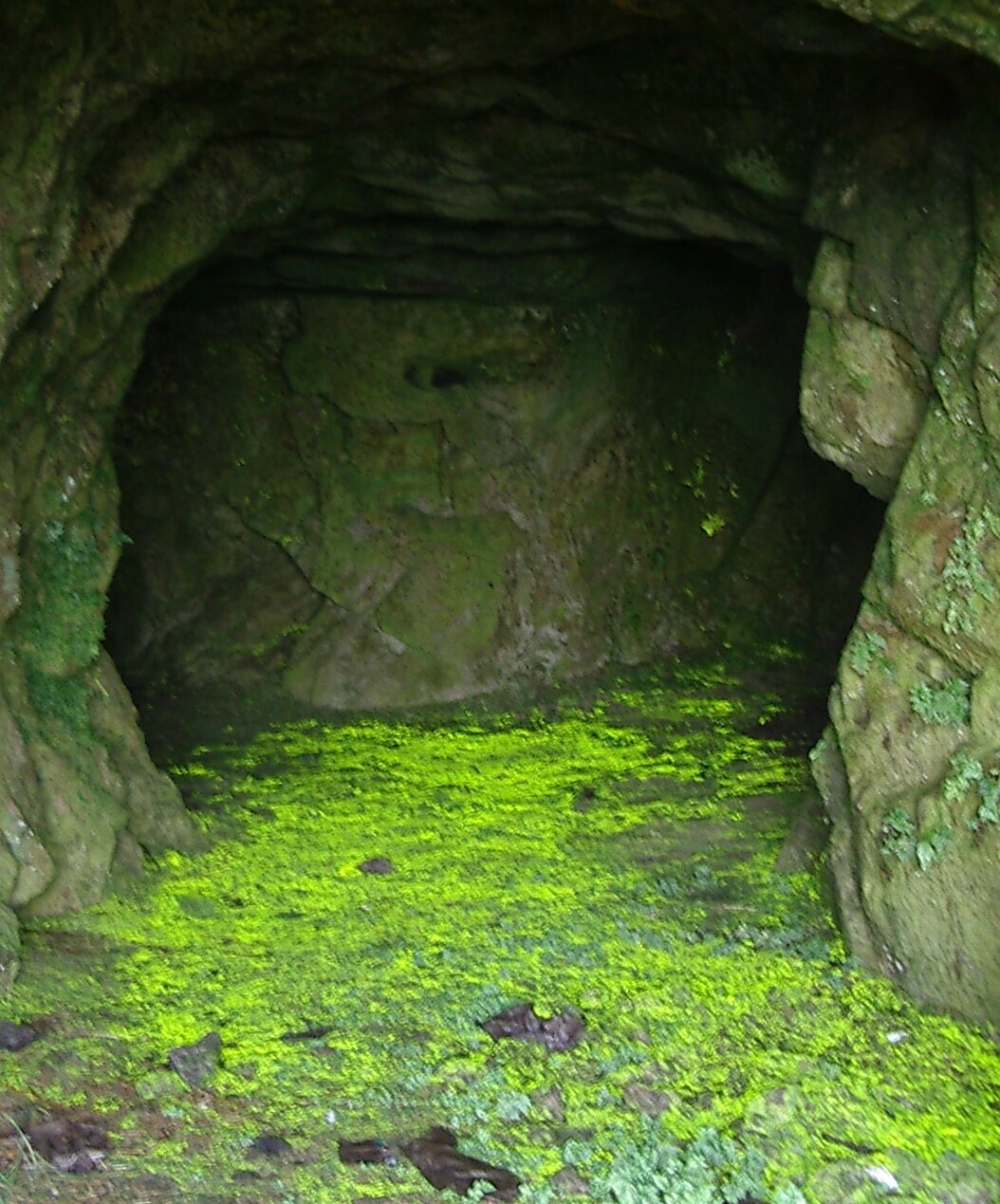This detailed color photograph captures the enigmatic mouth of a cave. The cave, predominantly dark, is framed by a vivid, almost neon green moss that carpets the ground and parts of the rugged granite and dark brown stone walls, giving a stark contrast to the otherwise shadowy setting. The entrance is arched, with the cave's walls extending upward and forming two distinct paths—one leading to the left and the other to the right—both veiled in darkness, making it impossible to see what lies beyond. The moss, which also clings to sections of the cave walls, appears luminous and even tree bark-like in some areas, adding to the textured appearance of the cavern. There are a few scattered leaves on the ground, contributing a natural touch to the scene. No animals or people are present, and there are no signs of writing, buildings, or vehicles within this vivid image, focusing solely on the intricate beauty of the natural cave environment.